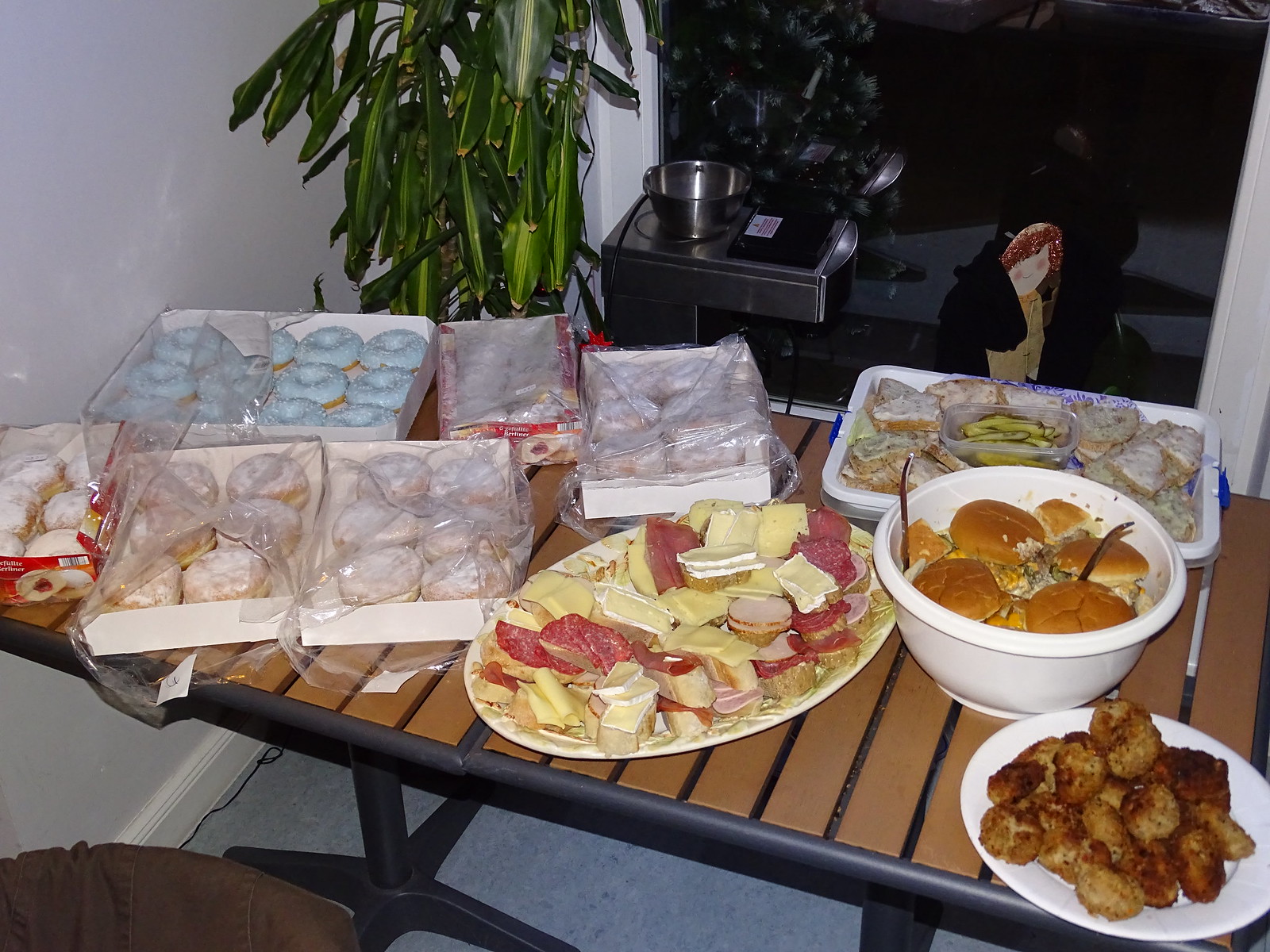This detailed photograph, taken indoors, captures a night-time setting indicated by the dark, windowed backdrop displaying a glass reflection. The focus is a landscape-oriented slat-top wooden table, edged in black with twin black pedestal legs. The table is laden with an eclectic array of party food, resembling a smorgasbord. Positioned in a room corner adorned with a potted plant and possibly a TV screen, the table also neighbors an espresso machine and a small stand-up angel figurine.

At the forefront is a vibrant display of various foods, beginning with a platter of charcuterie featuring an assortment of meats, cheeses, and breads. This is flanked by a plate of ambiguous fried items. A bowl of sliced pickles and what appears to be hamburger buns atop a salad with a couple of spoons are next in line. There's also a tray bearing frosted turnovers or sandwiches, and another bowl filled with what looks like cheesy pepper canapés or meatballs.

Dominating the scene are multiple boxes of donuts—each a feast for the eyes. These boxes, some white and some reddish, contain an assortment of donuts: blue-frosted, white-powdered, and jelly-filled varieties, with some appearing to be traditional Polish Paczkis. These treats are notably placed in plastic bags, with one box visibly torn open for easy access. A smaller box with a picture of a donut and a larger box of blue-frosted donuts stand out prominently.

In the left-hand corner, a chair is partially visible, rounding out the warm, inviting composition of this indoor celebration.